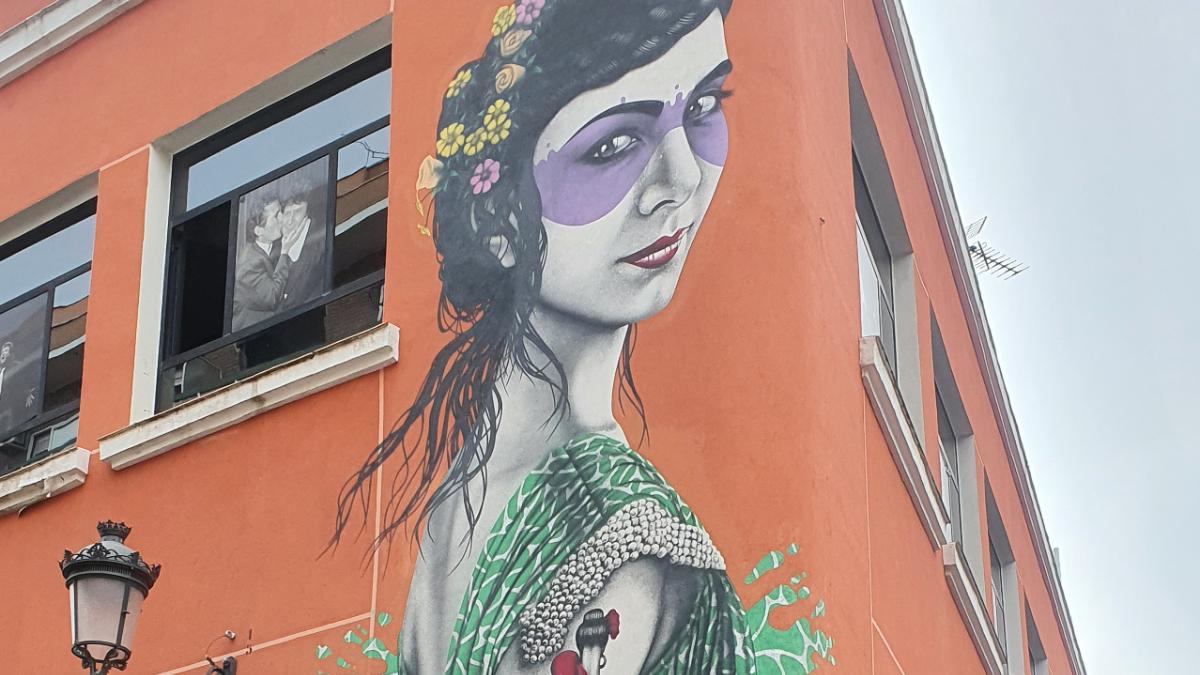This full-color photograph, taken outdoors during the day, captures the corner of an orange stucco building against a clear blue sky. Occupying the center-right of the image, an old TV antenna rises into view, while the lower left-hand corner features a streetlamp. The main focal point is an elaborate painting of a woman on the side of the building. She has dark brown hair adorned with flowers and wears a green dress accented with white details and beadwork on the sleeves. Her visage is striking, with a purple eye mask and bright red lips. A distinctive tattoo of a red lady adorns her bicep. The top floor of the building showcases windows, one of which displays a black-and-white picture of two men kissing, a common image in Sicily, hinting at the possible location. The photograph beautifully blends elements of urban artistry and architectural detail, creating a vivid and dynamic composition.